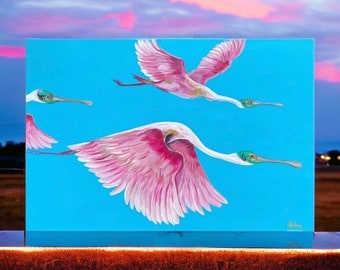This is a detailed photograph of a rectangular painting, centered in the frame, placed on a low, thin ledge made of a transparent, glossy material. The painting itself is also rectangular, with the top and bottom sides twice as long as the left and right sides. It features a solid light blue background and depicts three birds in mid-flight. These birds have white bodies, long white feathered necks, and are distinguished by their large yellow spoonbill-type beaks and green spots on their faces. Their wings are mostly pink with white tips. Notably, one bird is only partially visible, showing just its head. At the very bottom right of the painting, the artist's signature is delicately inscribed in yellow cursive text. The image appears to have been taken outdoors, as real clouds, a dark blue sky with hints of pink, brown grass, silhouetted tree lines, and ambient lights are visible in the background, adding a natural and somewhat atmospheric context to the scene.